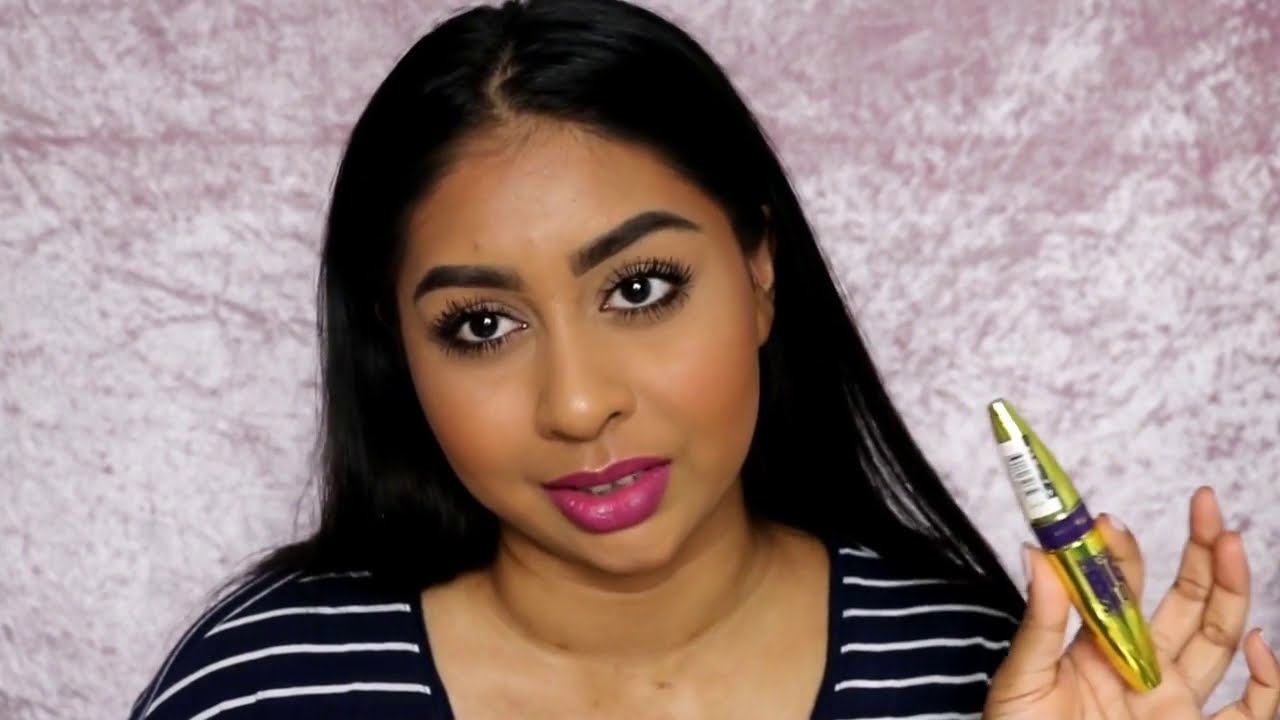A centered image features a woman, possibly Indian or Latina, against a pinkish textured marbled background reminiscent of a makeup store setting like Sephora. Her caramel complexion is complemented by her pink lipstick and striking black hair. She wears a black, white-striped V-neck shirt. In her left hand, held between her thumb and index finger, she holds a gold and purple eyeliner tool, still bearing a white barcode, suggesting it's a sample product. With her head cocked slightly to the right and one eyebrow raised, her expression appears ready to speak, exuding a sense of modeling or promotion. She is also characterized by her meticulous makeup, highlighted by prominent mascara.